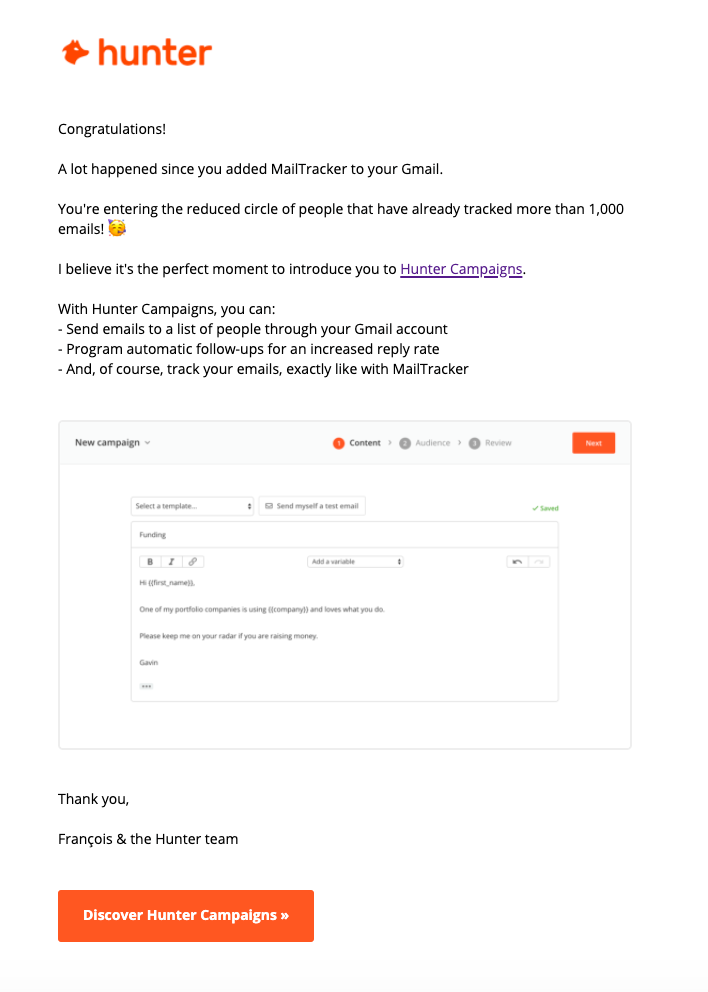The image is a screenshot featuring an announcement with an orange and white logo that includes the name "Hunter," possibly accompanied by an image of a wolf or a dog. The prominent text reads "Congratulations" and celebrates the recipient’s achievement of tracking more than 1,000 emails since integrating Mally Tracker with their Gmail account. An emoji of a party blower is included to mark the celebration.

The message introduces "Hunter Campaigns," written in purple and functioning as a clickable hyperlink. Hunter Campaigns allows users to send emails to a list of people via their Gmail account, schedule automatic follow-ups to boost reply rates, and track their emails similarly to Mally Tracker.

Additionally, the image contains a white box that resembles a new campaign interface. Below this, there is a message from "Franzis and the Hunter team." At the bottom, an orange rectangle with white text invites the viewer to “Discover Hunter Campaigns,” accompanied by a double right arrow icon.